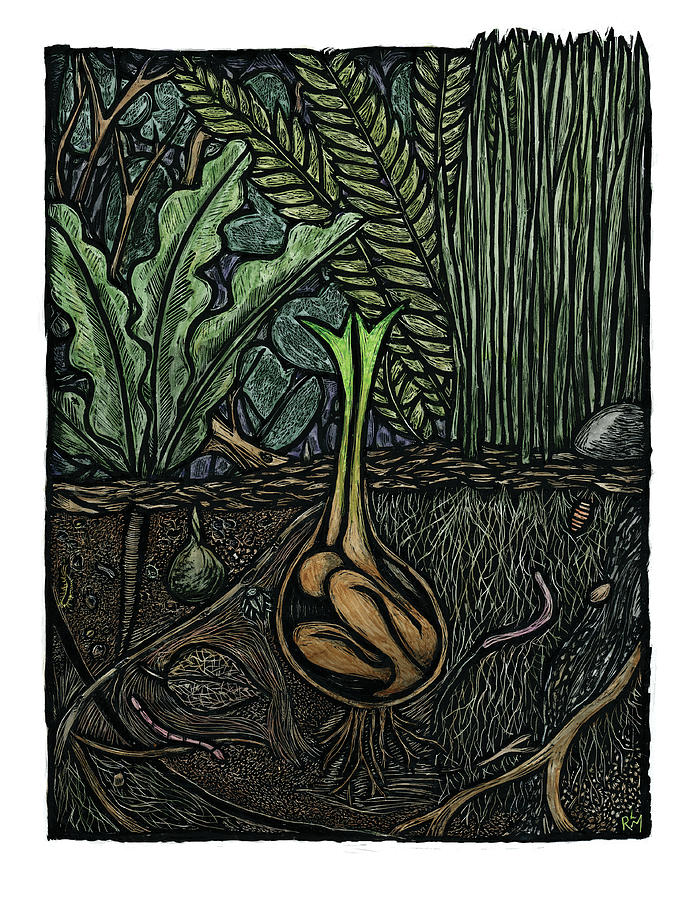The image is an intricate, abstract representation of plant life emerging from the ground, incorporating elements of both organic growth and human form. The upper section of the composition features a diverse array of foliage, including grass blades, loosely shaped leaves, and intertwining branches in shades of green. These plants seem to symbolize various types of flora such as dandelions, ferns, and perhaps wheatgrass.

Beneath the surface, the artwork reveals a complex network of roots and earthy elements. Among these subterranean details are several distinct items: a carrot and an onion embedded in the soil, occasional worms on the left side, and a peculiar leafy structure that doubles as a focal point.

The centerpiece of this artwork is a striking bud at the core, resembling a human figure curled into a fetal position. This figure appears to be the source from which the greenery sprouts, with arm-like extensions growing upward, integrating the human form into the botanical motif. The overall color palette is dominated by subdued tones—grays, dark wood hues, and muted greens—accentuating the impression of growth and rebirth emerging from the earth.